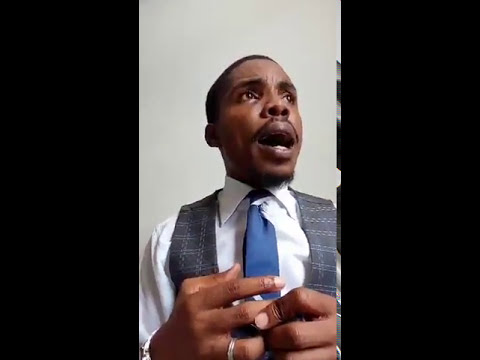The image features a well-dressed black man positioned directly in the center against a white background. He appears to be indoors, perhaps in a professional setting taken during the day. The man is looking off to the top right side of the image with a wide open mouth and a face that conveys shock or disturbance, his eyes slightly watery. He has very short black hair, black eyebrows, a thin black mustache, and some black hair on his chin. He is wearing a white collared button-up shirt with a blue tie and a gray vest adorned with white dotted lines running horizontally and vertically. His hands, positioned at the bottom of the image, are clutched together, and he wears a silver ring on one of his fingers. The background of the image is unadorned except for some black rectangles on the left and right sides.